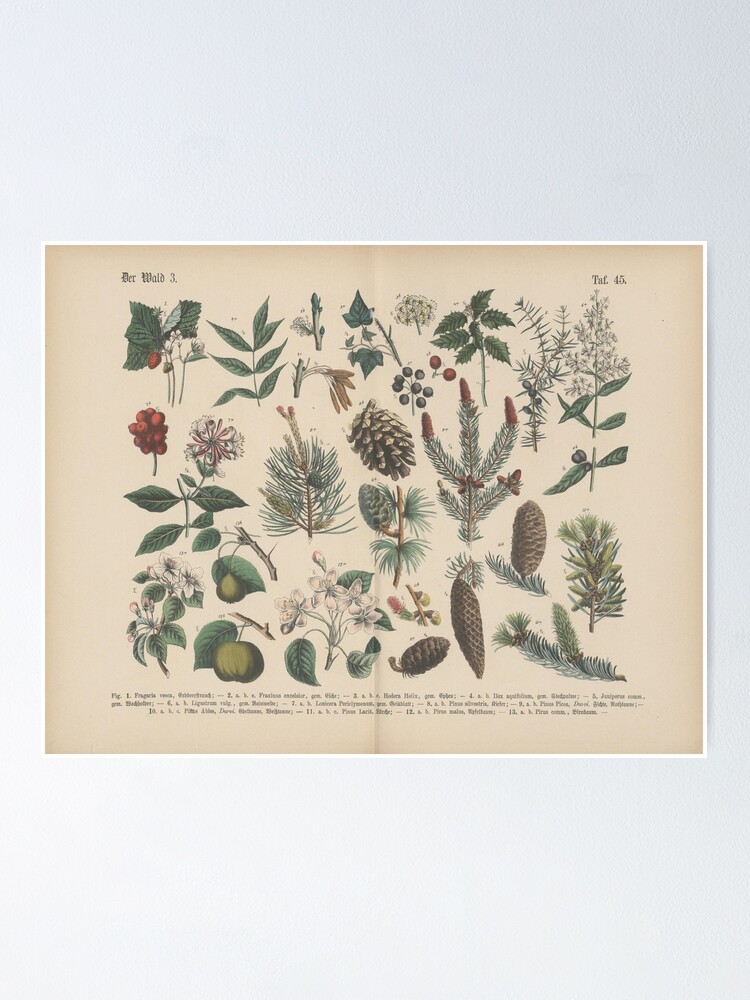This richly detailed poster is an old-fashioned ink illustration reminiscent of Currier and Ives' work, depicting a diverse collection of natural elements you might find hanging from trees. The illustration features various pinecones—including at least two distinct types—branches adorned with pine needles, and an assortment of leaves, berries, and fruit. The botanical elements seem randomly distributed across the page, creating a visually intricate collage. At the top left of the poster, the word "DERWALD" is elegantly scripted in a fancy font, while "TAFF45" is displayed at the top right. Each botanical item is accompanied by numbers, and a legend at the bottom of the page corresponds to these numbers, providing detailed identification.